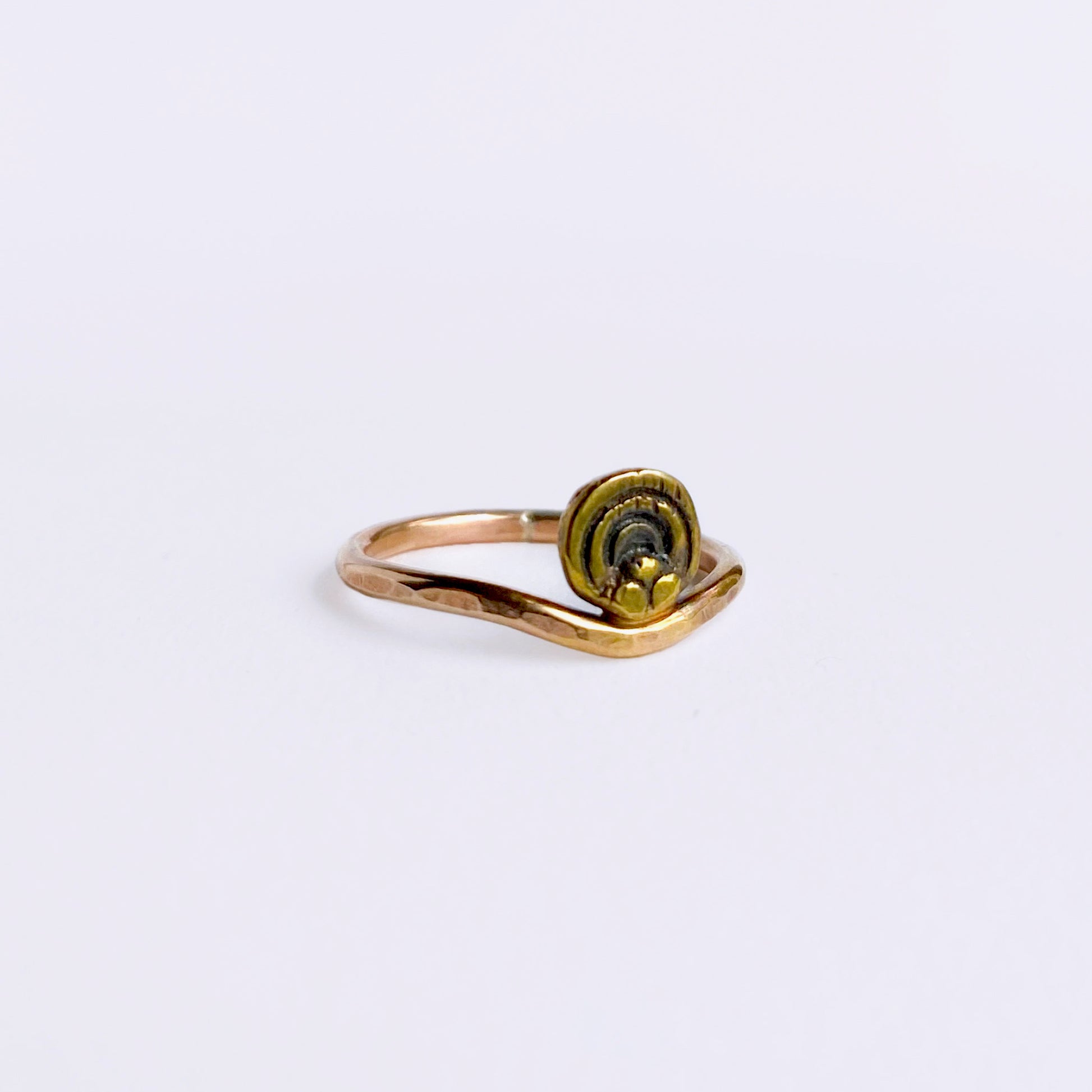This close-up photograph showcases a ring resting on a slightly grey-tinged white background. The ring itself exhibits a primarily golden hue with subtle copper tints, suggesting it could be made from gold or a gold-like alloy, such as brass. The craftsmanship of the ring appears imperfect and primitive, with an asymmetrical shape and various curves that create a curvy triangle at the base. The surface features slight grooves, adding to its frail and delicate appearance, possibly indicating it is designed for a woman or a young girl.

At the center of the ring, where you might typically find a gemstone, there is a unique circular symbol, composed of three smaller gold circles or blobs at the bottom. These elements spread out into a pattern of concentric circles featuring darker ridges on the exterior, giving the impression of a layered, intricate design. A reflection of a black object is also noticeable on the left-facing side of the ring. This detailed and somewhat enigmatic symbol, cast in dull grey and gold tones, adds a mysterious and artisanal touch to the ring's overall aesthetic.